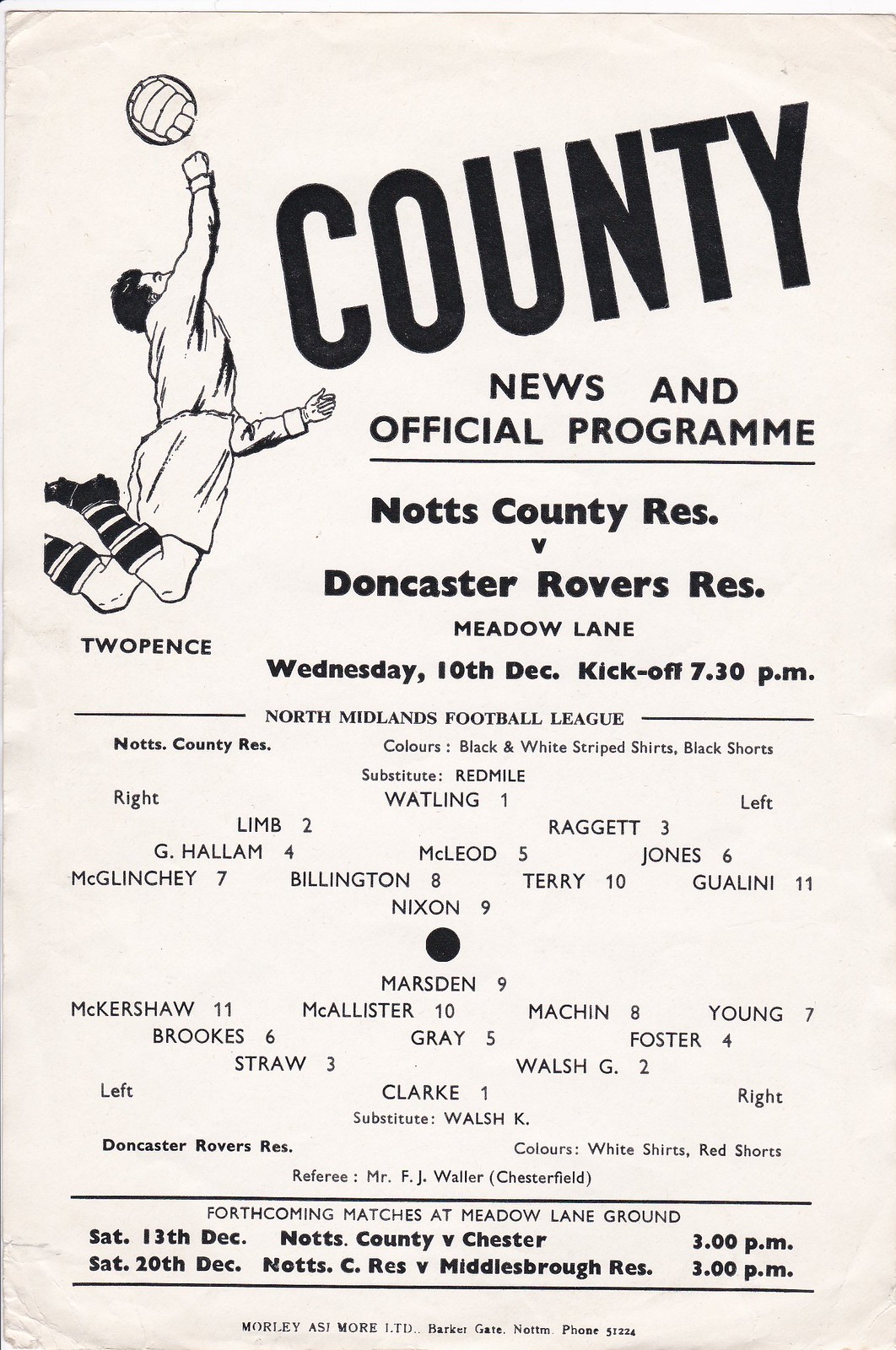This black and white print features a page from an old soccer program, set against a beige background. The header reads, "County News and Official Program," highlighting the match between Knotts County R.E.S. and Doncaster Rovers R.E.S. at Meadow Lane, scheduled for Wednesday, 10th December, with a 7:30 p.m. kickoff, priced at 2 pence. A hand-drawn graphic of a soccer player in mid-air, attempting to head a ball, embellishes the top left corner. The main text lists player details for both teams, including numbers and positions, with Knotts County R.E.S. donned in black and white striped shirts with black shorts. The referee, Mr. F.J. Waller from Chesterfield, is also named. Towards the bottom, upcoming matches at Meadow Lane Ground are mentioned: Knotts County versus Chester on Saturday, 13th December at 3 p.m., and Knotts County R.E.S. versus Middleborough on Saturday, 20th December at 3 p.m. Additional text includes printers' details and contact information.